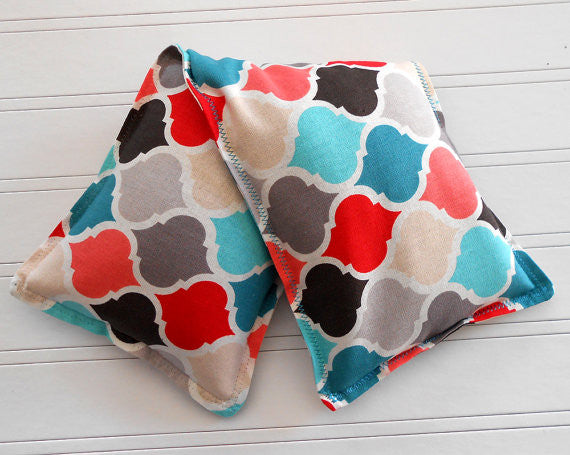The image depicts a hand-sewn or machine-sewn multi-colored pillow or heating/cooling pack, filled with materials like rice for temperature control. The object is designed to be placed on the body for therapeutic purposes, such as alleviating pain or providing comfort, with its shape appearing to be long and folding to fit the frame. The color pattern on the cushion includes shades of red, gray, cream, blue, black, and tan, and the threading is teal. This multi-use pack is displayed on a white striped wooden bench or table background.